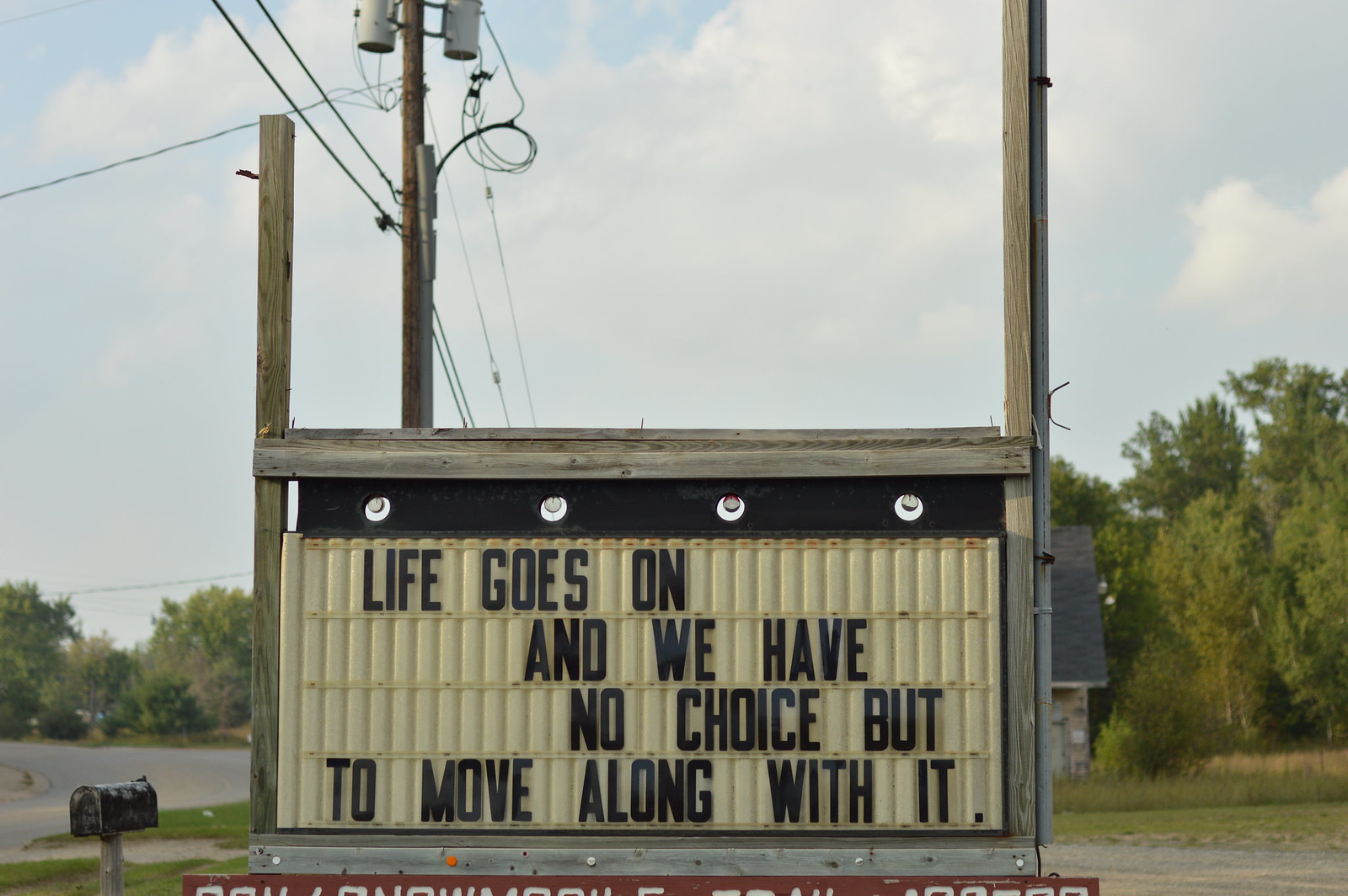In this detailed outdoor daytime photograph, the lower half prominently features a white marquee sign with black lettering arranged in four lines: "Life goes on," "and we have," "no choice but," "to move along with it." Above the marquee is a rectangular black strip adorned with four evenly spaced light bulbs, unlit, against a wooden frame. Two posts, one on each side, support the sign. In the background to the left stands a vertical brown utility pole with electrical lines extending from it and two mounted transformers. Trees and a blue sky with scattered clouds form the backdrop, while the curved road edges to the left. In the lower left foreground, a weathered black mailbox on a wooden post can be seen. Further below the main text of the sign, partially obscured, are white letters on a red background. The surrounding scene suggests a tranquil local setting, possibly near a residential area or a small business.